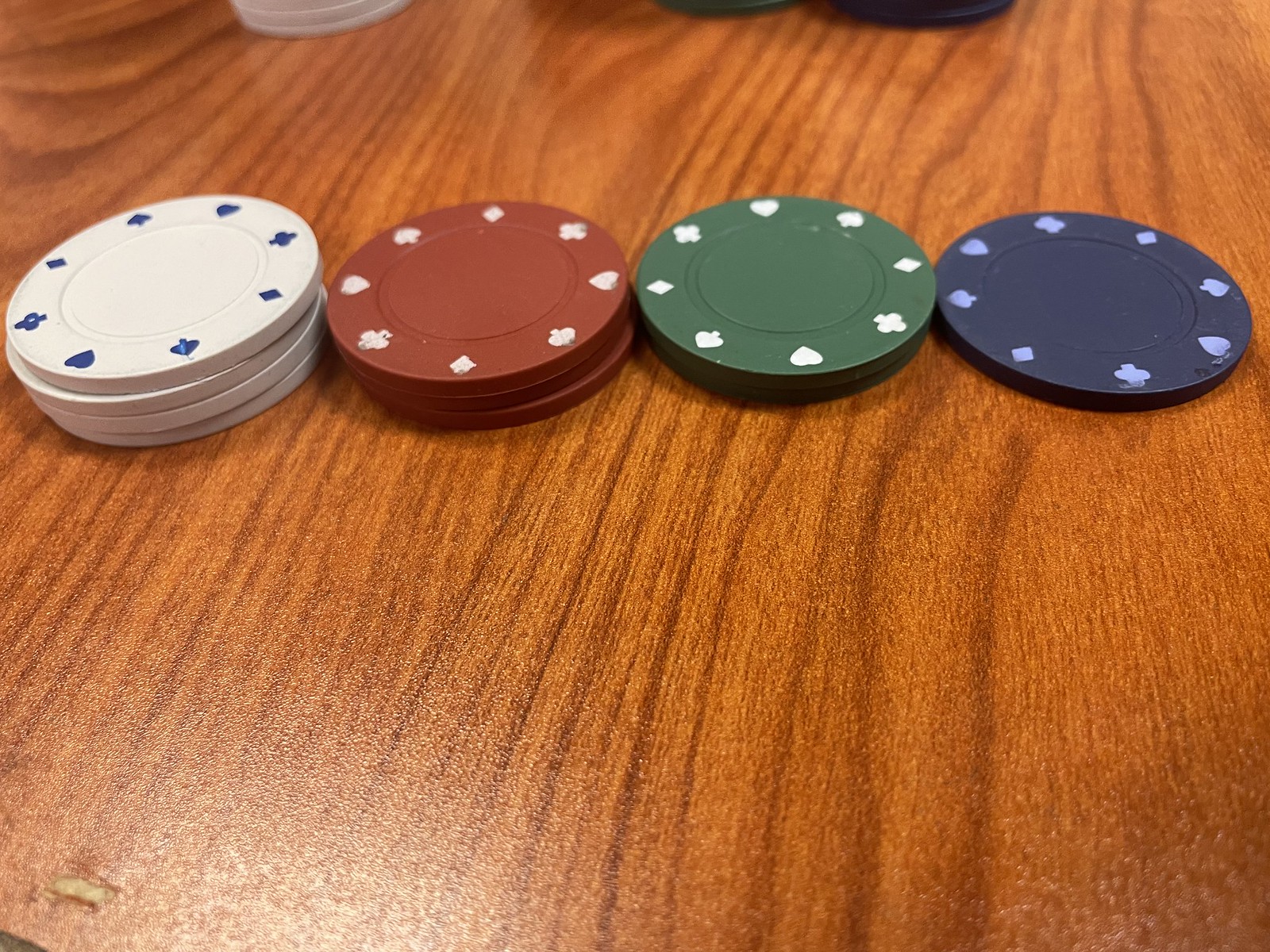In this photograph, there are four meticulously arranged stacks of poker chips displayed horizontally from left to right. The leftmost stack comprises four white poker chips adorned with small blue emblems etched around their edges. Next to them, the second stack consists of three red poker chips, each featuring white edging. The third stack holds two green poker chips, distinguished by white symbols along their sides. The final stack on the right contains a single blue poker chip with subtle bluish symbols on its edges.

The table surface underneath the chips is a reddish oak hue, accented by vertical brown lines that add a textured appearance. Notably, in the bottom left-hand corner, there's a small imperfection in the wood, a minor blemish or cut. The poker chips are precisely laid out in a single horizontal line, creating a clear visual progression: four chips, three chips, two chips, and one chip, adding up to a total of ten poker chips—four white, three red, two green, and one blue.

At the top edge of the photograph, there are additional smaller sections of poker chips, though the exact number is indeterminable due to the reduced visibility. These sections include hints of white, blue, and possibly green chips, but the tops of these stacks are out of view, making it difficult to ascertain their exact count.